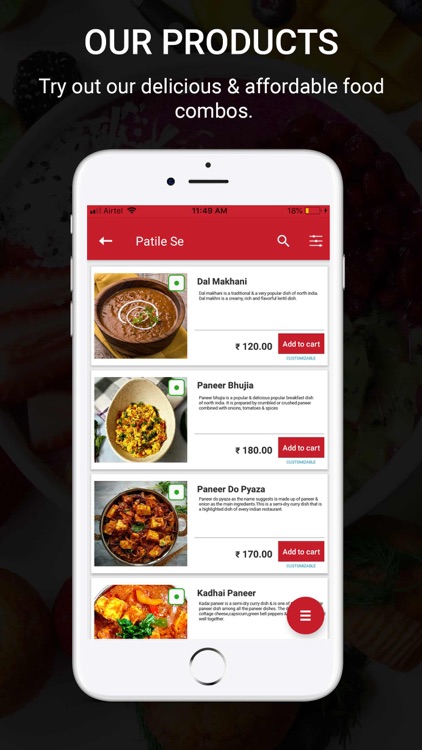This advertisement features a sleek, portrait-oriented black rectangular box with a promotional message that reads: "Our Products: Try our delicious and affordable food combos." Central to the image is a generic smartphone displaying a storefront app for a restaurant. The app interface showcases various appetizing dishes, specifically traditional Indian recipes. Highlighted items include Dal Makhani, Paneer Bhujia, Paneer Do Pyaza, and Kadai Paneer, all of which can be added to the cart for a seamless ordering experience. The smartphone screen has been digitally enhanced to illustrate the ease of browsing and selecting meals through their app.